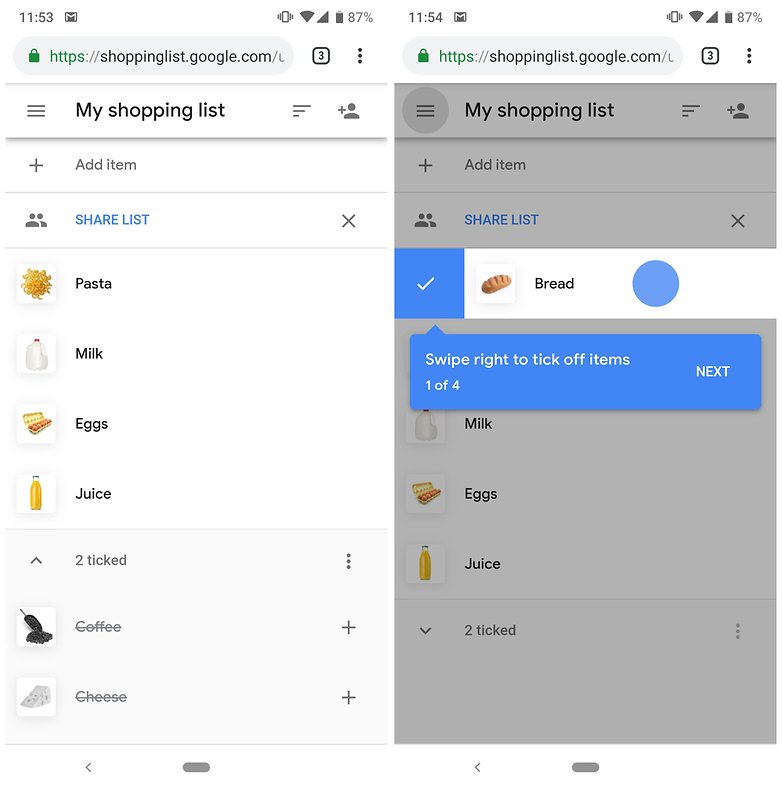The image consists of two side-by-side screenshots taken a minute apart from a shopping list website on Google. 

**Left Screenshot (Timestamp: 11:53 AM):**
- **Top Bar:**
  - Gmail notification icon.
  - Phone signal icon with bars.
  - Wi-Fi symbol.
  - Battery indicator showing 87%.
- **Web Address:** `http://shoppinglist.google.com`
- **Header:** 
  - A square icon with the number "3".
  - Three vertical dots (menu icon).
  - "My Shopping List" displayed in a black font on a white bar.
- **Icons:**
  - Gray cartoon head and shoulders icon indicating a user menu.
- **Main List:**
  - **"Add Item"** section with a gray plus sign.
  - **"Share List"** option in blue text, flanked by an "X".
  - **Categories with Images and Items:**
    - **Pasta:** Picture of a yellow pasta pile, labeled "pasta" in black.
    - **Milk:** Image of a milk jug with a red cap, labeled "milk" in black.
    - **Eggs:** Yellow carton with orange eggs, labeled "eggs" in black.
    - **Juice:** Glass bottle of orange juice labeled "juice" in black.
    - **Coffee:** Image of coffee beans with a gray strikethrough, labeled "coffee"; includes a gray plus sign.
    - **Cheese:** Gray block of cheese, labeled "cheese"; includes a gray plus sign.

**Right Screenshot (Timestamp: 11:54 AM):**
- **Top Bar:**
  - Same icons as the left screenshot, including 87% battery and "3" icon.
- **Web Address:** `http://shoppinglist.google.com`
- **Header:** Identical to the first screenshot.
- **Main List:**
  - **"Add Item"** section.
  - **"Share List"** option.
  - **Highlighted Category:** "Bread"
    - White box with a blue and white checkmark.
    - Picture of a brown loaf of bread.
    - Blue circle indicator.
    - Blue pop-up message with white text: "Swipe right to take off items 1 of 4".
  - **Repeating Items:**
    - **Milk:** Same image of a milk jug with a red cap.
    - **Eggs:** Image of the same yellow carton with orange eggs.
    - **Juice:** Same glass bottle of orange juice.
    - **Note:** Two items ticked off.

Both screenshots show detailed views of a digital shopping list with visual icons, images, and item categories, alongside interface elements for adding and sharing the list.